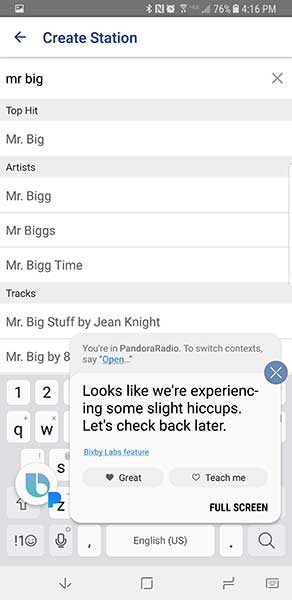A cell phone screenshot captured at 4:16 PM with a 76% battery level displays the "Create Stations" page. The screen features various icons at the top and a faint gray line under the "Create Stations" header positioned towards the left. Below the line, "Mr. Big" is listed, followed by "Top Hit." Continuing downward, "Mr. Big" is again listed under the "Artist" section, this time with an extra 'G' as "Mr. BIGG." Further down, "Mr. Biggs" appears, with the addition of an 'S,' spelled "Mr. BIGGS." Underneath is "Mr. Big Time" where "Big" is written as "BIGG." The "Tracks" section lists "Mr. Big Stuff" by Gene Knight, where "Knight" is spelled "K-N-I-G-H-T." A pop-up box on the screen reads, "Looks like we’re experiencing some slight hiccups. Let’s check back later," offering an option to click for full screen.